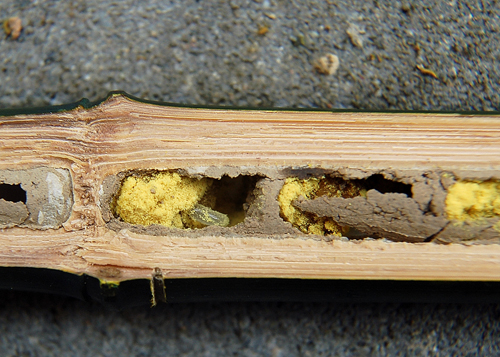The photograph showcases a close-up view of a horizontally cut piece of termite-infested wood, positioned against a gray, textured background that resembles gravel or sandy beach. The wood reveals a cross-section displaying several chambers within it. These chambers vary in composition: some are packed with yellow, sawdust-like material and others filled with a mixture of green chunks, brown clay-like substances, and gunk. The wood's exterior features a distinct, jet-black border, contrasting sharply with the light, pale wood grain that runs horizontally from left to right. Four primary chambers are visible, each with mottled, damp wood surrounding them. The photograph captures the intricate and damaged internal structure of the wood, indicative of an advanced termite infestation. Small flecks of leaves and debris scattered around the wood further emphasize its natural, decayed state.